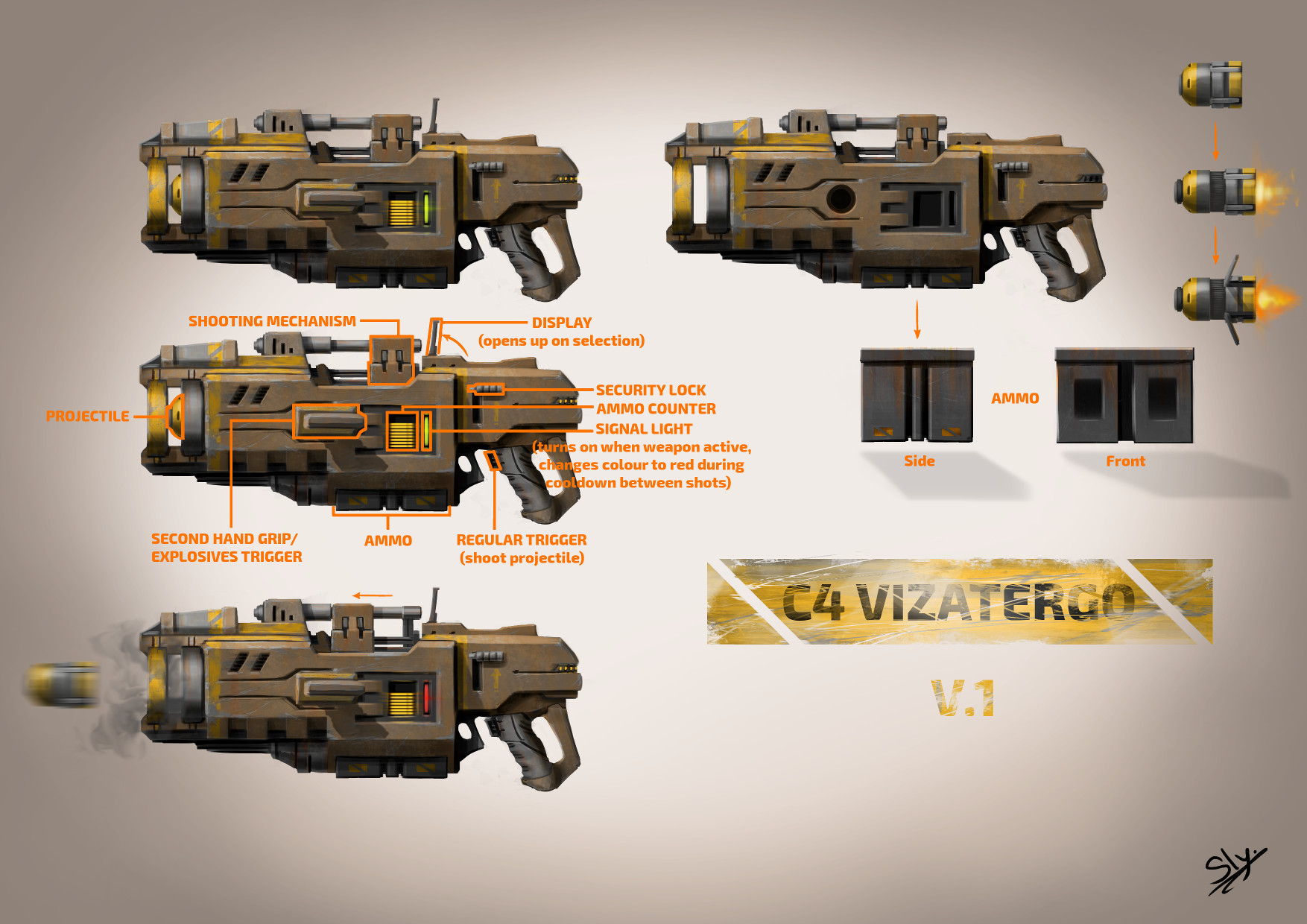The illustration showcases a detailed concept art of a gun named "C4 Visa Turbo Version 1," signed by the artist "SLY" in the bottom right corner. The artwork comprises four primary images, each providing a different perspective and informational overlay of the weapon. The main image at the top center displays the gun facing left, emphasizing its robust design with brown, gray, and yellow accents, suggestive of a grenade or rocket launcher. 

Below it, there’s a comprehensive labeled diagram, identifying key components such as the shooting mechanism, second hand grip, explosives trigger, and the display which opens up on selection. The projectile, depicted as a small C4 cartridge, is also highlighted. 

A third image captures the gun in action, firing a C4 cartridge, where an explosion and the projectile are both visible, while in the lower left, the gun is shown without a projectile loaded.

On the right-hand side of the illustration, there are detailed sequential visuals of the C4 cartridge: initially normal, then impacted, and finally as it exits the gun. Additionally, there are illustrations of the ammunition boxes marked "C4."

The background of the concept art is a gradient of light to medium brown, with a brighter center spotlighting the gun. Despite the digital medium, the level of intricate details reflects advanced concept design, potentially for a video game.